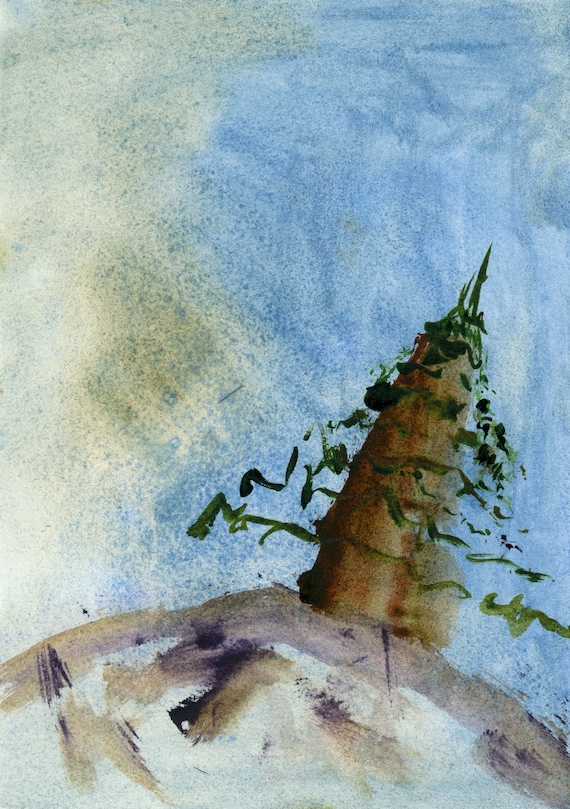The image is an abstract watercolor painting. On the right side, a blue sky fades into a lighter, cream-colored sky on the left, giving an impression of sunlight. The bottom of the painting features a rounded, maroon and brown mound, possibly a hill or rock, with patches of white and hints of purple. Perched on this mound is a structure resembling a narrow lighthouse or castle tower, brown in color with black squiggly lines. The structure tilts slightly to the left and is enveloped in olive-green, streamer-like shapes, which seem to sprout from and surround it, adding a sense of movement. The painting has a soft, muddied texture with no sharp edges, rendering it a subtle and undefined piece of art.